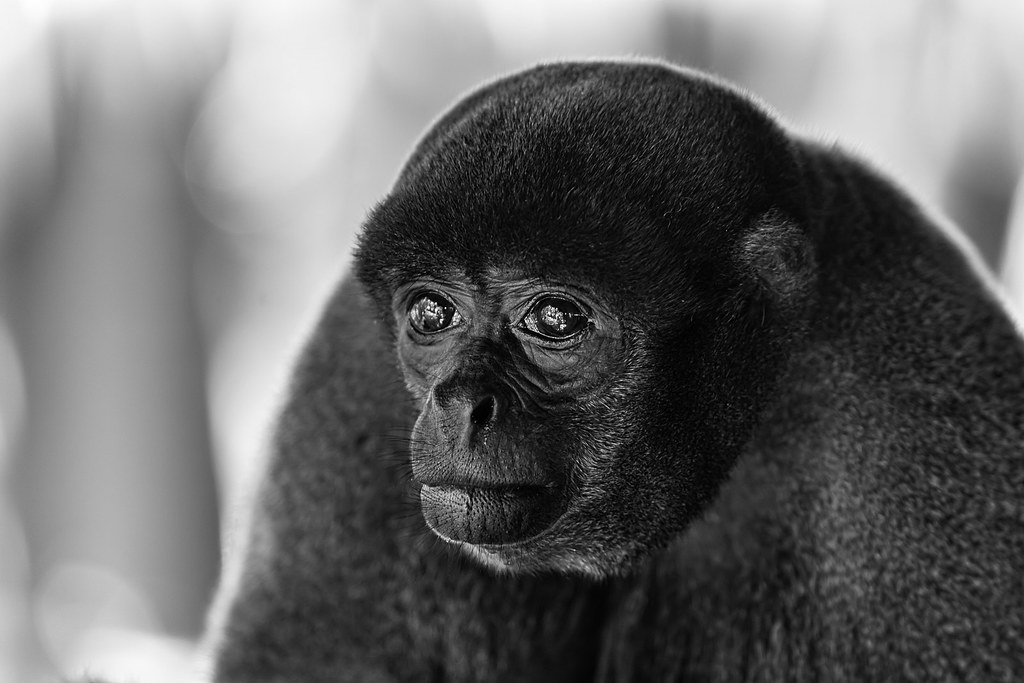This detailed black-and-white photograph captures a baby ape, possibly a small monkey, in a highly focused and poignant moment. The image zeroes in on the ape's face, showcasing the intricate details of its black fur, deeply expressive eyes, and wrinkled, skin-like features around its nose and mouth. The reflection in its large, dark eyes adds a layer of depth to the photo. The ape, situated in the center or slightly to the right, appears pensive and at peace, staring directly into the camera. Its left ear is visible, and the texture of its fur, especially the fuzz on top of its head, is meticulously detailed. Moving away from the face, the fur on its body becomes less sharp, eventually blending into a completely blurred background of white, gray, and black hues. The background, indistinct and almost glowing, contrasts with the sharpness of the primate's face, adding to the ethereal quality of the photograph.